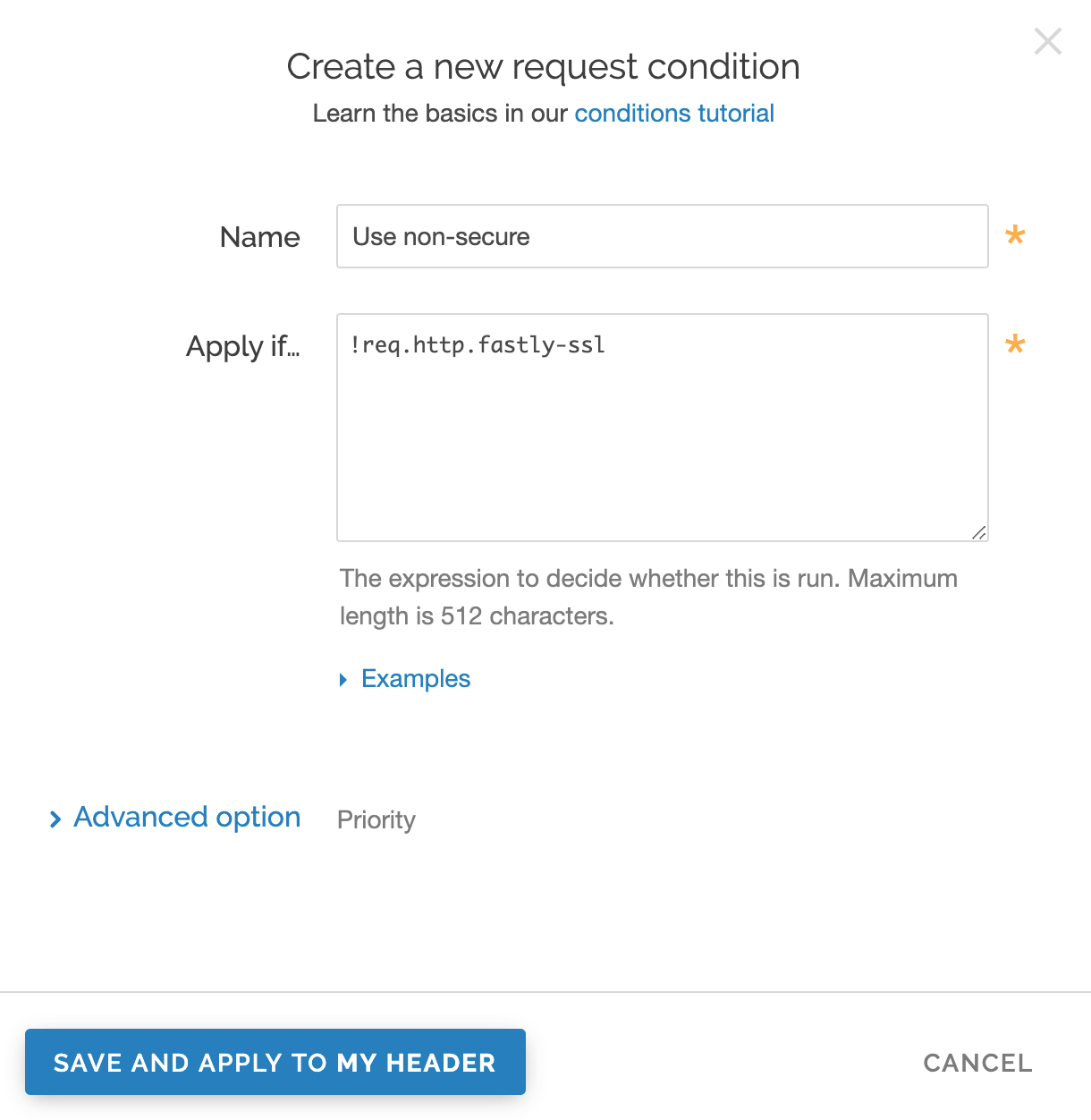The image features a clean, white background with a prominent heading in the largest font that reads "Create a New Request Condition." Just below the heading, a subtitle encourages users to "Learn the basics in our Conditions Tutorial," with the "Conditions Tutorial" phrase highlighted in blue.

The image showcases two input fields available for user entry. The first input field is labeled "Name" and includes a checkbox option labeled "Use Non-Secure." The second input field, which appears larger, is labeled "Apply If." Both input fields have an orange asterisk on their right-hand side, likely indicating required fields.

At the very bottom of the screen, there is a blue button labeled "Save and Apply to My Header," with white text. In the lower right-hand corner of the image, a "Cancel" option is displayed for user convenience. Additionally, the image features blue clickable text that reads "Examples" and "Advanced Options," suggesting further resources or settings available to the user.